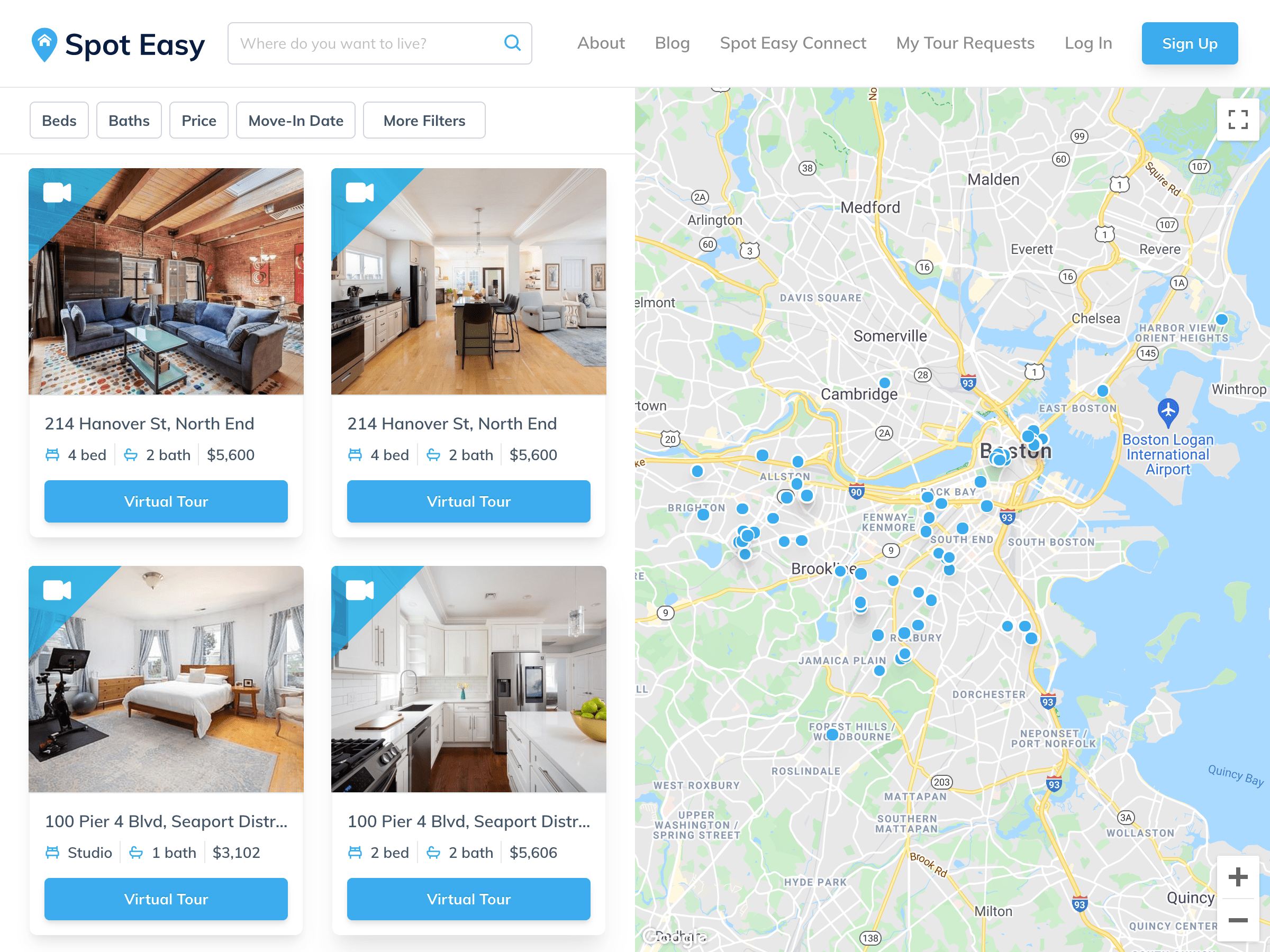A detailed screenshot depicts the user interface of the SpotEasy website, set against a clean white background. Dominating the top section is the SpotEasy logo beside a search bar adorned with a blue magnifying glass icon. Below the search bar are navigation options including "About," "Blog," "SpotEasy," "Connect," "My Tour Request," and "Login," followed by a prominent blue "Sign Up" button.

On the main part of the page, a map of Boston is displayed, dotted with several blue location markers. To the left of the map, a sidebar features a series of gray rectangles which contain various search filters: "Beds," "Baths," "Price," "Move-in Date," and "More Filters." Each filter option displays neatly within its respective rectangle.

Embedded within the sidebar are four smaller squares, each showcasing thumbnails of different properties. Each thumbnail has a camera icon in its corner, indicating the option for visual content. One highlighted property, featuring an interior image which resembles a cozy log cabin, is listed at 214 Hanover Street, North End, with specifications of four bedrooms, two bathrooms, and a price of $5,600. A blue rectangle labeled "Virtual Tour" in white text is prominently displayed below the listing.

Additionally, another property listed at 100 Pier 4 Boulevard in the Seaport District features similar details, including four bedrooms and two bathrooms, with partial text indication "DISTR..." completing the description. Each property maintains the consistent feature of a blue "Virtual Tour" button, allowing prospective renters to view the interiors remotely.